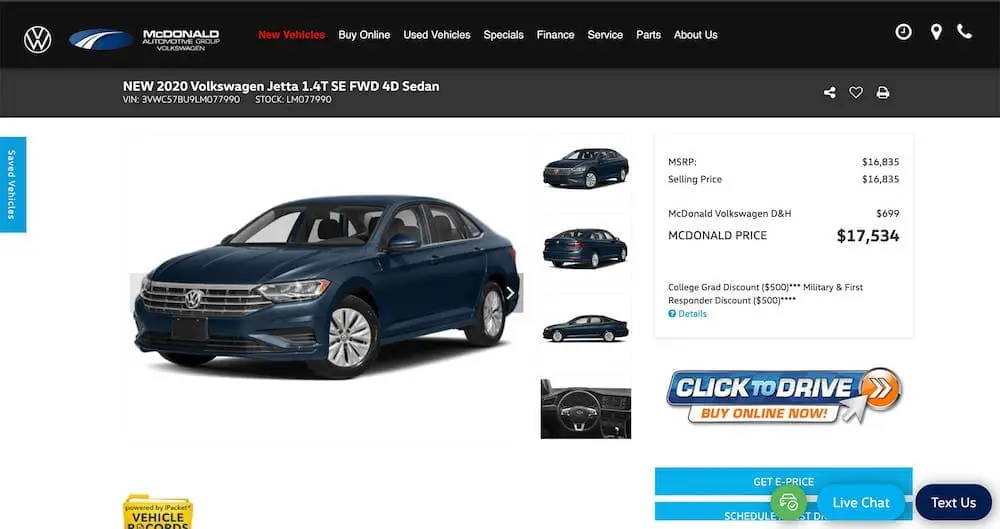This image depicts a promotional page from a car dealership associated with McDonalds, featuring a logo of BW Dealers in the top left corner. The layout includes various navigation headings such as "Buy Online," "Used Vehicles," "Specials," "Finance," "Service," "Parts," and "About Us." Prominently displayed beneath these headings is an image of the new 2020 Volkswagen Jetta 1.4T SE FWD 4D sedan. The car, showcased in a dark blue color, is accompanied by multiple high-quality pictures highlighting its sleek design and solid aluminum or stainless steel wheels. The total price listed for the vehicle is $17,534. Additional information is provided, although the text is small and somewhat difficult to read. A call-to-action prompt encourages potential buyers with "Click to Drive. Buy Online Now," situated above a blue button for live chat or text support for any further questions.